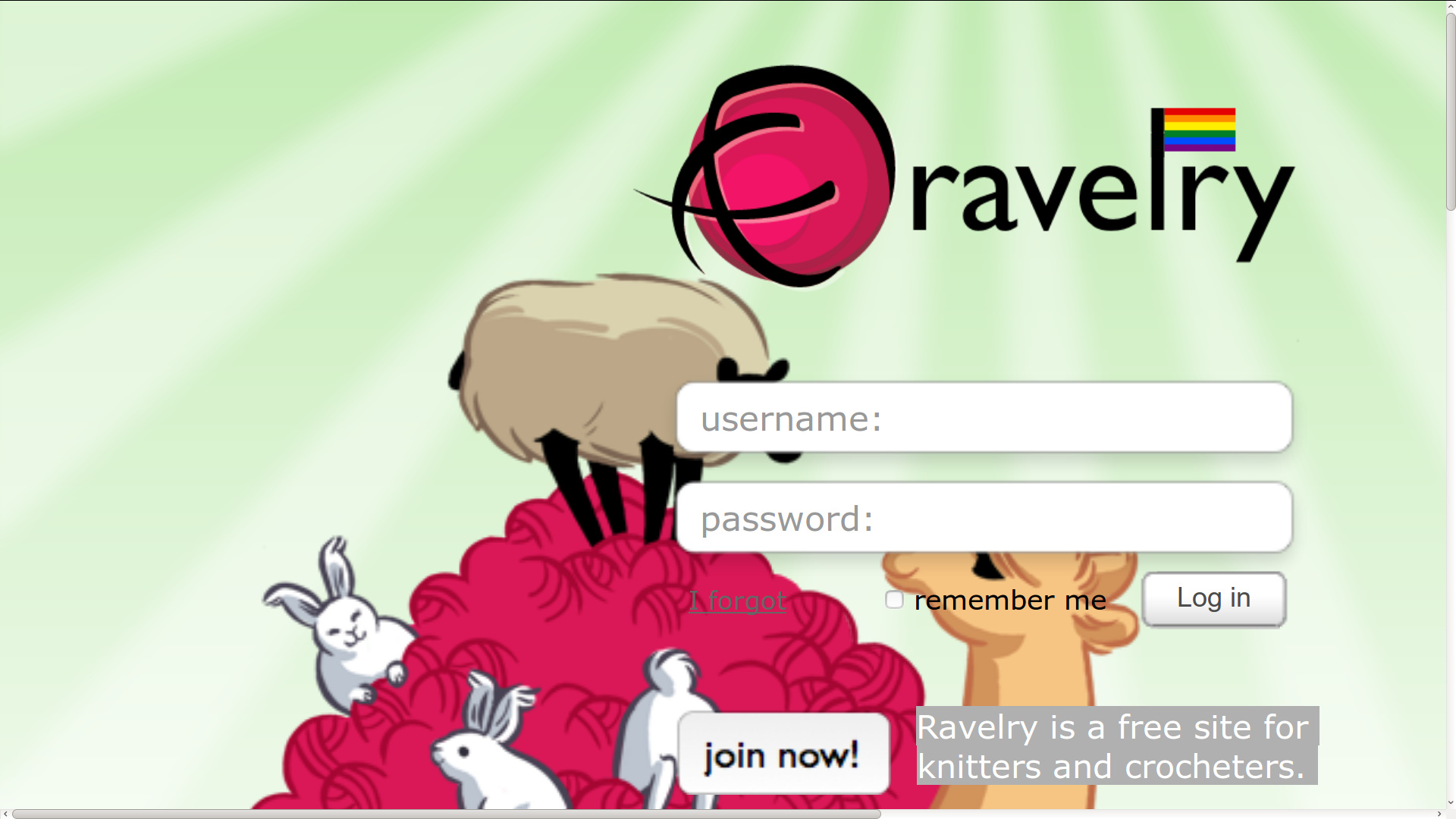A detailed screenshot capture taken on a laptop or desktop computer features a browser interface with evident scroll bars on the right and bottom of the image, indicating a traditional computing setup. Displayed on the screen is a login page for a website named FRAVELRY, although the exact name is obscured by a stylized design. A prominent red sphere serves as the background for the site's title, which is wrapped around it, making the exact lettering difficult to discern. A noteworthy detail is the stylized letter "L," adorned with a rainbow flag, symbolizing the pride flag.

The login interface comprises fields for entering a username and password. Beneath these fields, there is a login button, flanked by a "Remember Me" checkbox and an "I forgot" password recovery link. Lower on the page, a "Join Now" button invites new users with a note stating, "Ravelry is a free site for knitters and crocheters."

Adding a playful and charming touch to the page, the background is adorned with a whimsical cartoon illustration. Here, bunnies, sheep, and an alpaca stand on a hill made of yarn balls, engaging each other in a cute and endearing manner. This scene is set against a green backdrop with white rays descending to emulate a sunrise, enhancing the website's friendly and inviting atmosphere.